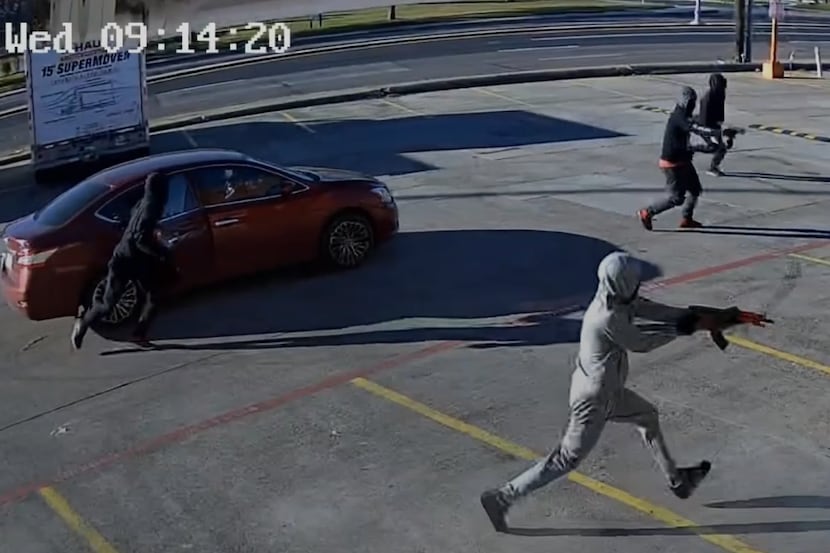The surveillance camera still frame, captured at 09:14:20 on a Wednesday, shows a tense scene unfolding in a parking lot. The image is rectangular, with the width being twice the length of the height, and features a light gray asphalt surface marked by yellow lines delineating parking spots and red lines designating a fire lane. In the center of the scene, a red four-door car, possibly a Nissan Altima, is positioned. A person in dark clothing is seen exiting the back right door of the car. To the right, three individuals dressed in hoodies, with their faces obscured, are charging forward, gripping firearms and assault rifles. The nearest figure to the camera sports a gray hoodie and pants, while the others are clad in black. The background reveals a U-Haul truck parked to the left, enhancing the sense of urgency. The whole area appears brightly lit, casting clear shadows, indicative of a sunny day. This detailed frame suggests an imminent shootout in the parking area.